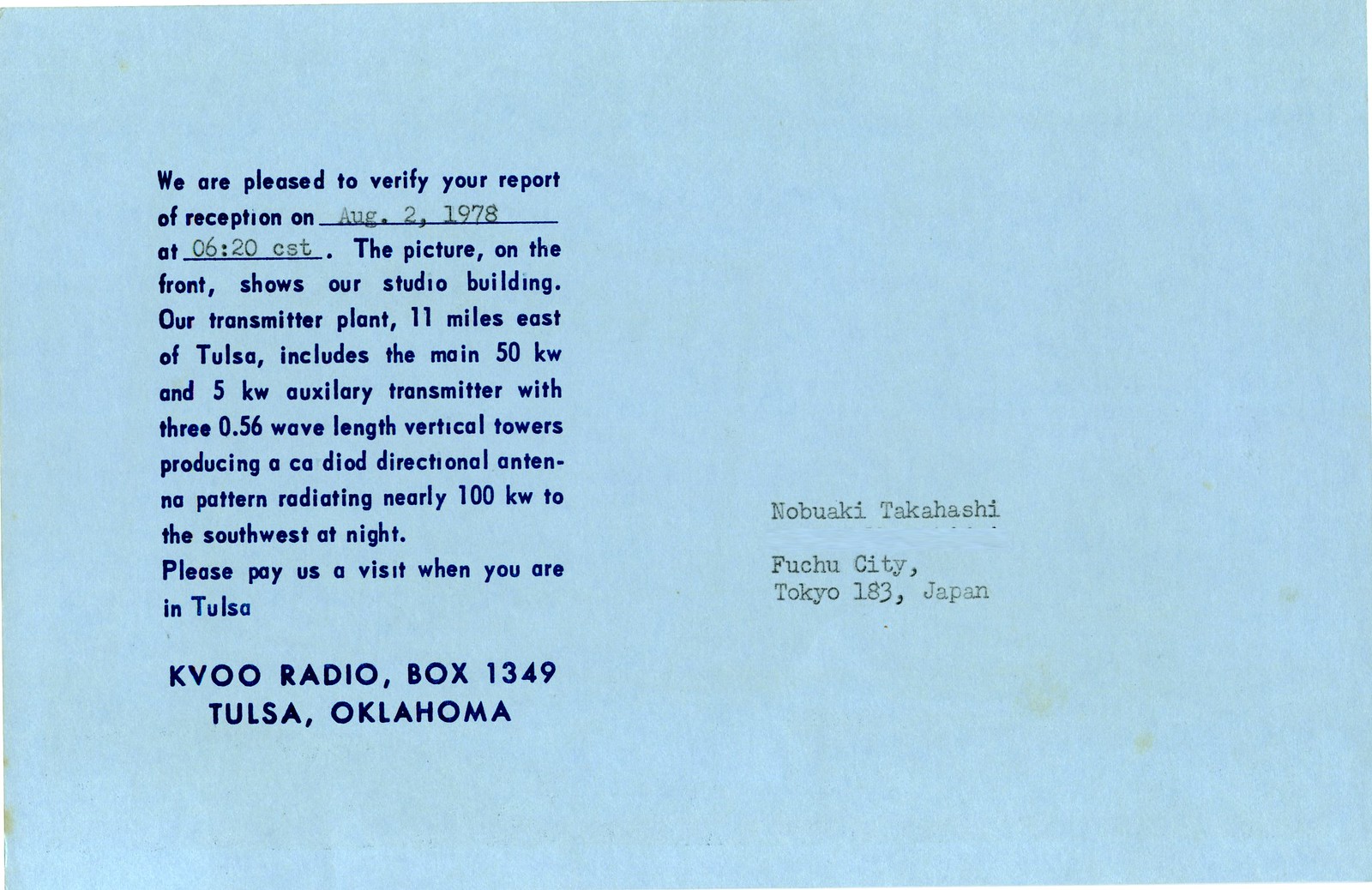This image depicts a blue reception report verification card sent to Nobuaki Takahashi, residing in Fuchu City, Tokyo 183, Japan. The card confirms the receipt of a report of reception on August 2, 1978, at 0620 CST. On the front, a picture showcases their studio building. The card details that the transmitter plant, located 11 miles east of Tulsa, includes a main 50 kW and an auxiliary 5 kW transmitter, with three 0.56-wavelength vertical towers. These towers produce a CA diode directional antenna pattern, radiating nearly 100 kW to the southwest at night. A personalized note invites the recipient to visit the station when in Tulsa, and it is signed with the KVOO Radio Box, 1349 Tulsa, Oklahoma.